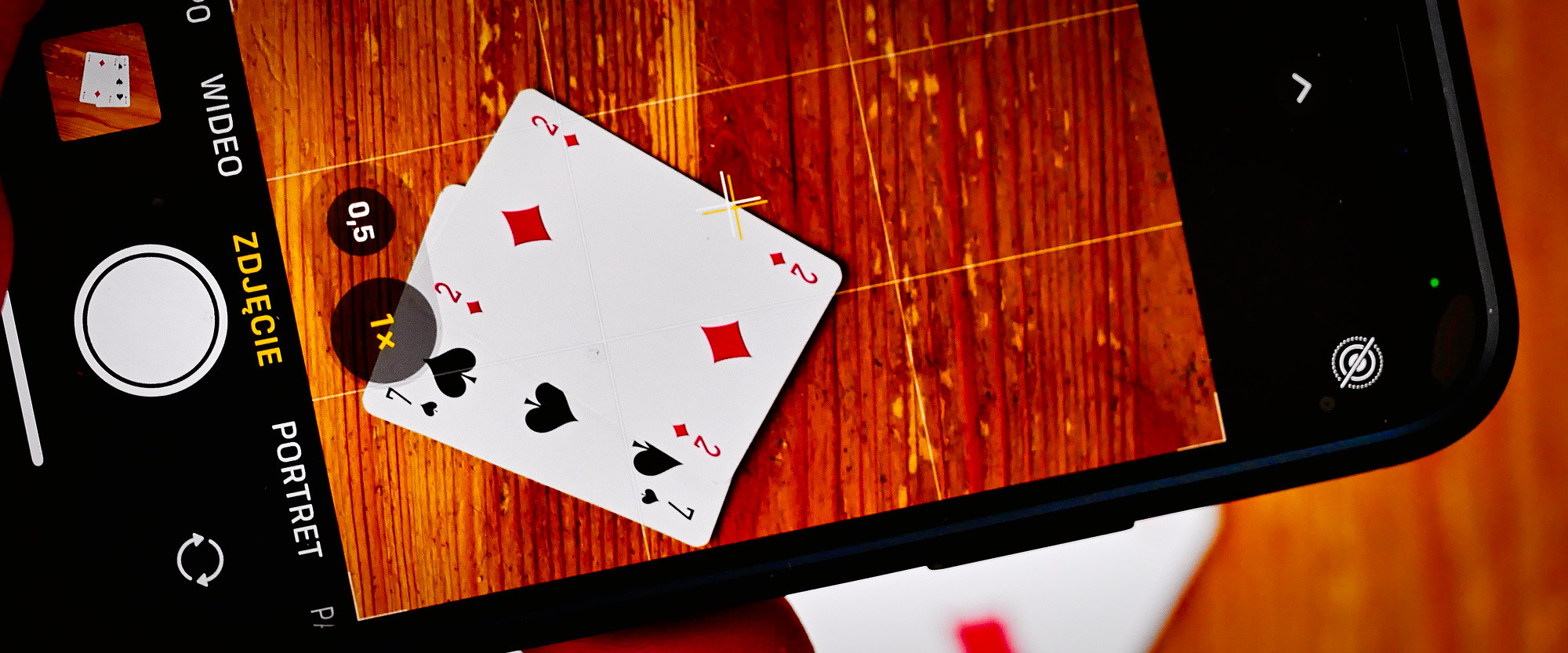In this image, a smartphone is seen in camera mode, attempting to capture a photograph of two playing cards placed on a wooden table: the two of diamonds and the seven of hearts. The phone's display shows the camera set to 1x zoom, which is the default setting. The interface language appears to be Polish, and a small crosshair is visible in the center of the screen for precise focusing and alignment. The bottom left corner of the display shows thumbnail previews, indicating that several photos of these cards have already been taken. The scene is well-lit, highlighting the texture of the wooden surface and the vivid colors of the playing cards.